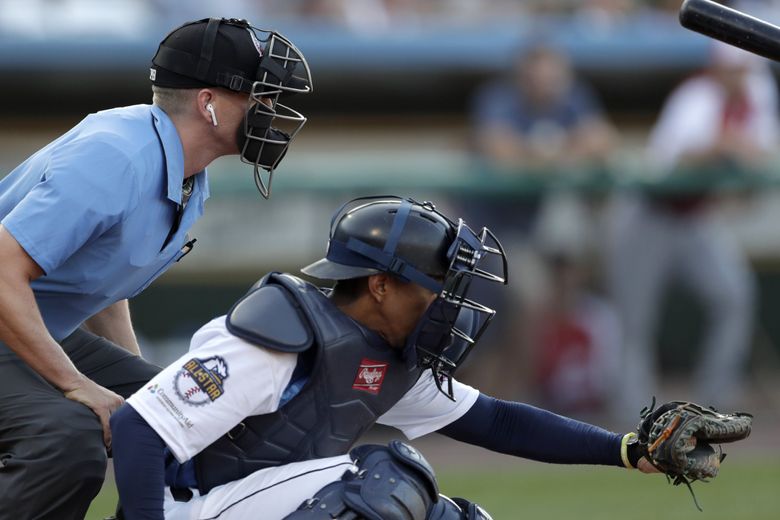In this highly detailed, up-close image from a high-definition sports camera at a baseball game, we see a side view of a catcher and an umpire. The catcher, situated to the right, is squatting and dressed in a white uniform adorned with blue lettering on the sleeve that reads "All-Star," along with a baseball stitching. He is wearing extensive dark blue padding for protection, including leg guards, and has a black hat and strapped mask covering his face. His left hand is extended, holding a catcher’s mitt.

Directly behind the catcher, the umpire is also squatted. He is clad in a light blue half-shirt paired with gray pants, which show the protruding impressions of knee cushions. The umpire has on a face mask, a black baseball cap, and an earbud in his right ear. The background of the image is blurred but reveals the green field, blurred players, and the audience in the stands. A black baseball bat is partially visible in the top right corner, suggesting the presence of a batter preparing for play.